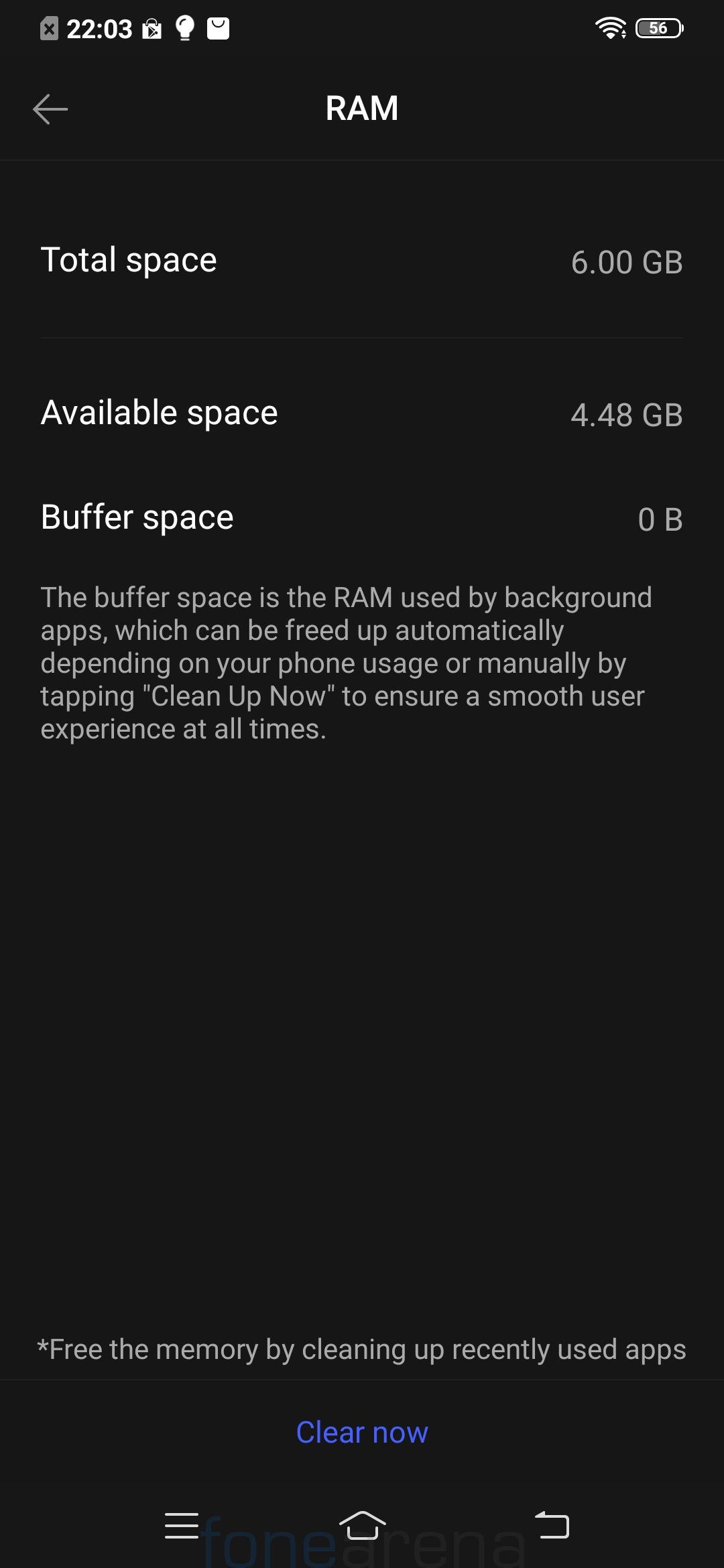The screenshot displays a smartphone's RAM status on a black screen with white font. At the center bottom, a blue button labeled "Clear Now" is prominently featured. The top left corner shows the time as 22:03 along with three icons: a right arrow, a light bulb, and an email icon. Adjacent to these, the Wi-Fi symbol is illuminated, and the battery indicator displays "56%."

Central to the screen is the word "RAM" with three categories listed beneath it. The first category, "Total Space," shows 6 gigabytes. The second category, "Available Space," indicates 4.48 gigabytes. The third category, "Buffer Space," reads 0 bytes, accompanied by a description explaining that the buffer space is used by background apps and can be freed up either automatically or manually to ensure smooth performance.

At the bottom, a starred message advises, "Free the memory by cleaning up recently used apps." Below this message, the "Clear Now" button appears in blue. Finally, three navigation icons are present at the bottom of the screen: three horizontal white bars on the left, a home screen icon in the center, and a back arrow on the right.